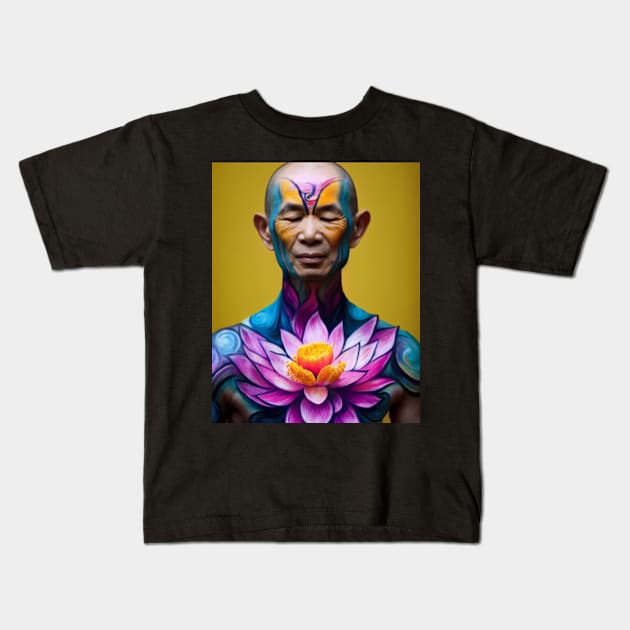This image showcases a black short-sleeved t-shirt with a regular collar, set against a stark grey background. The t-shirt features a detailed and vibrant depiction of an older Buddhist man, who appears to be meditating with his eyes closed and his shaven head adorned with intricate tattoos. The man's skin is predominated by blue-tinted tattoos that extend from his head down to his chest, blending with darker blue accents to create facial details. Covering his chest is a prominent lotus flower, vividly colored with shades of purple and orange, displaying wide-open petals. The lotus flower emerges from a dark blue background on the man's body, while his tattooed head features a mix of orange and blue relief swirly symbols. Despite the golden or brownish tint behind the man's image on the shirt, it stands out sharply against the dark black fabric of the t-shirt. Notably, the design on the shirt almost appears to be photoshopped for display purposes, reinforcing an artistic and striking visual impact.